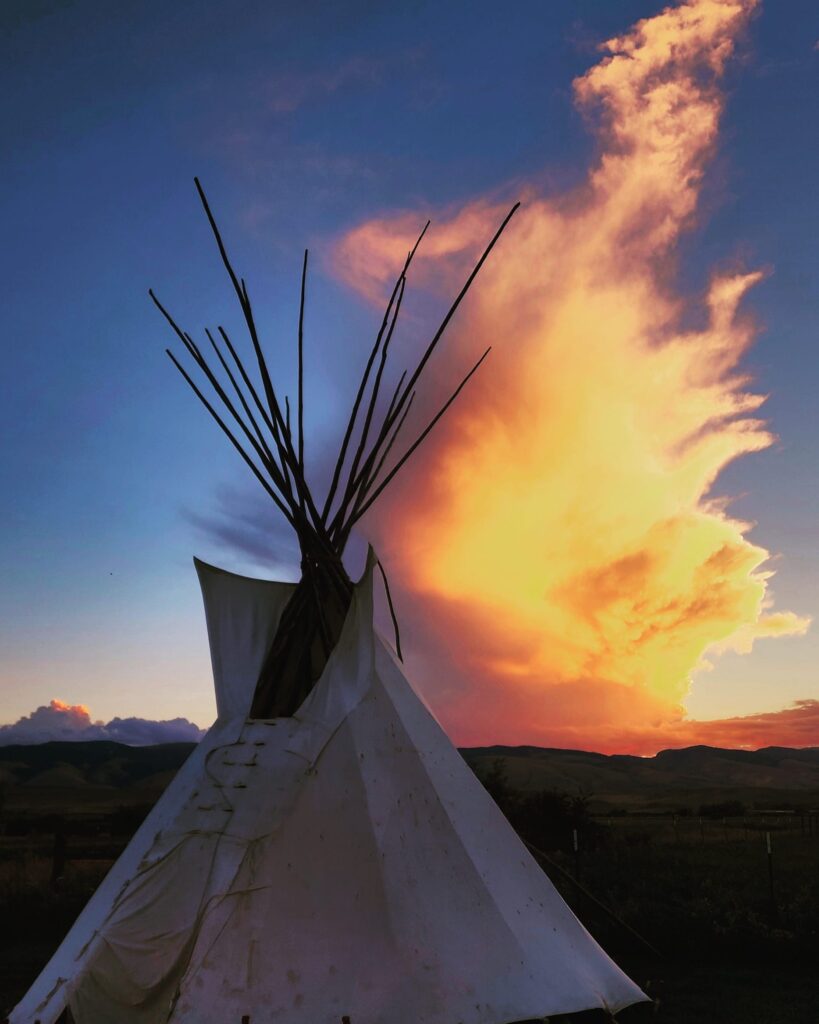This photograph captures a close-up view of a white teepee with closed flaps and white laces at its entrance, set against a Western sunset landscape. The teepee, possibly made of canvas or animal skins, is supported by a series of thin, brown sticks protruding at various angles from its top. The ground around the teepee is dark and indistinct, with some grass visible near its base. In the distance, slightly rolling hills and a faint fence can be seen. The sky is a deep blue, tinged with the vibrant colors of the setting sun. A prominent cloud formation stretches horizontally across the sky, transitioning from gray and white at the top to a bright orange-yellow near the horizon, with touches of violet-lavender on the left.